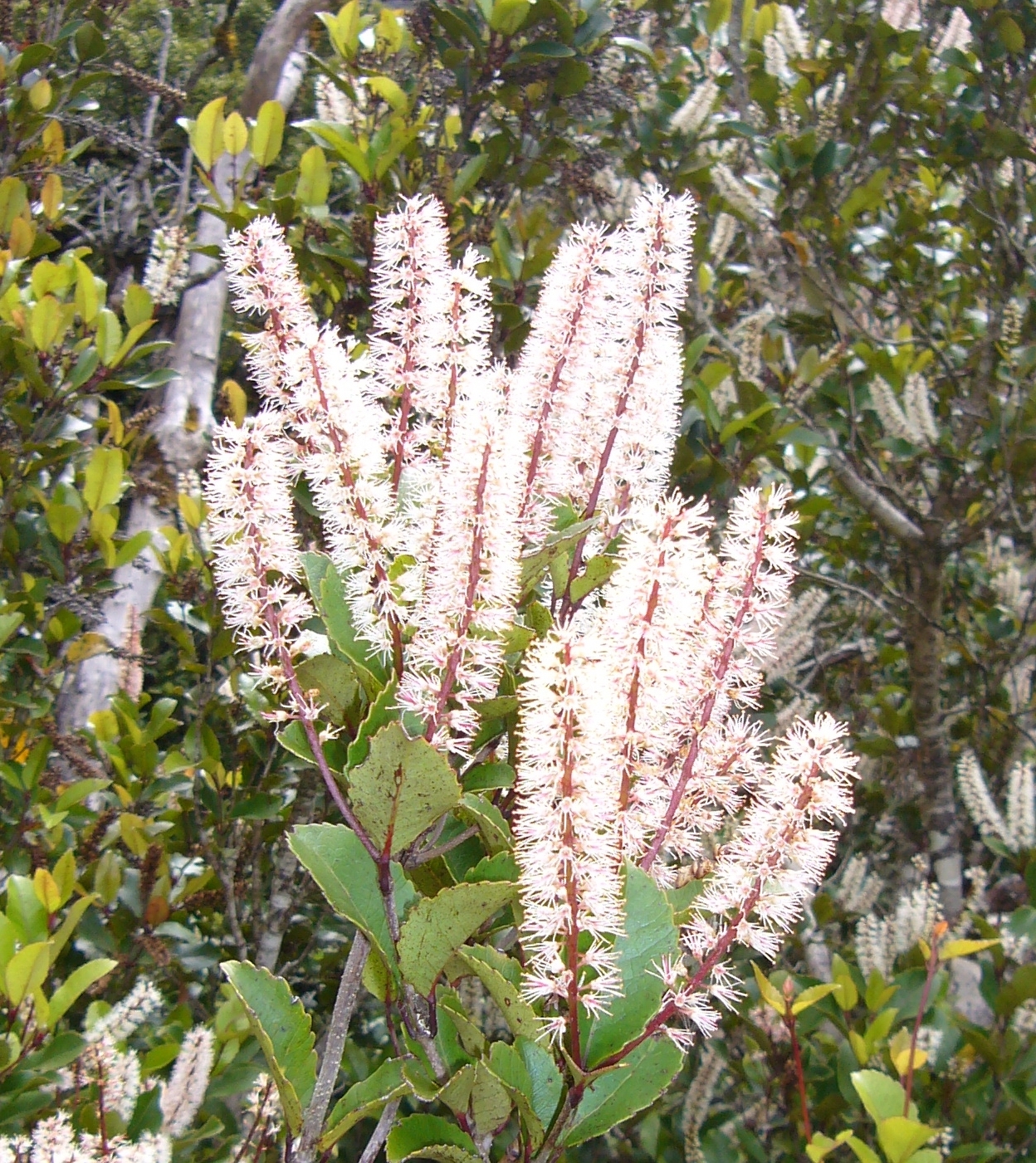The photograph captures a striking outdoor scene on a sunny day, focusing on an unusual, tall plant with white, delicate petals and pinkish hues. These flowers, arranged cylindrically, extend upward from rich, brown stems. Each petal appears like a delicate shard, contributing to the flower's distinctive and somewhat unusual vertical shape. Surrounding the flowers are large green leaves with jagged edges, which, in some areas, transition to a more yellowish tone. The background features light brownish-gray tree trunks and branches, slightly blurred, further emphasizing the plant's prominent, rich colors. The overall composition highlights the vibrant contrast between the white and pink flowers and the lush green foliage.